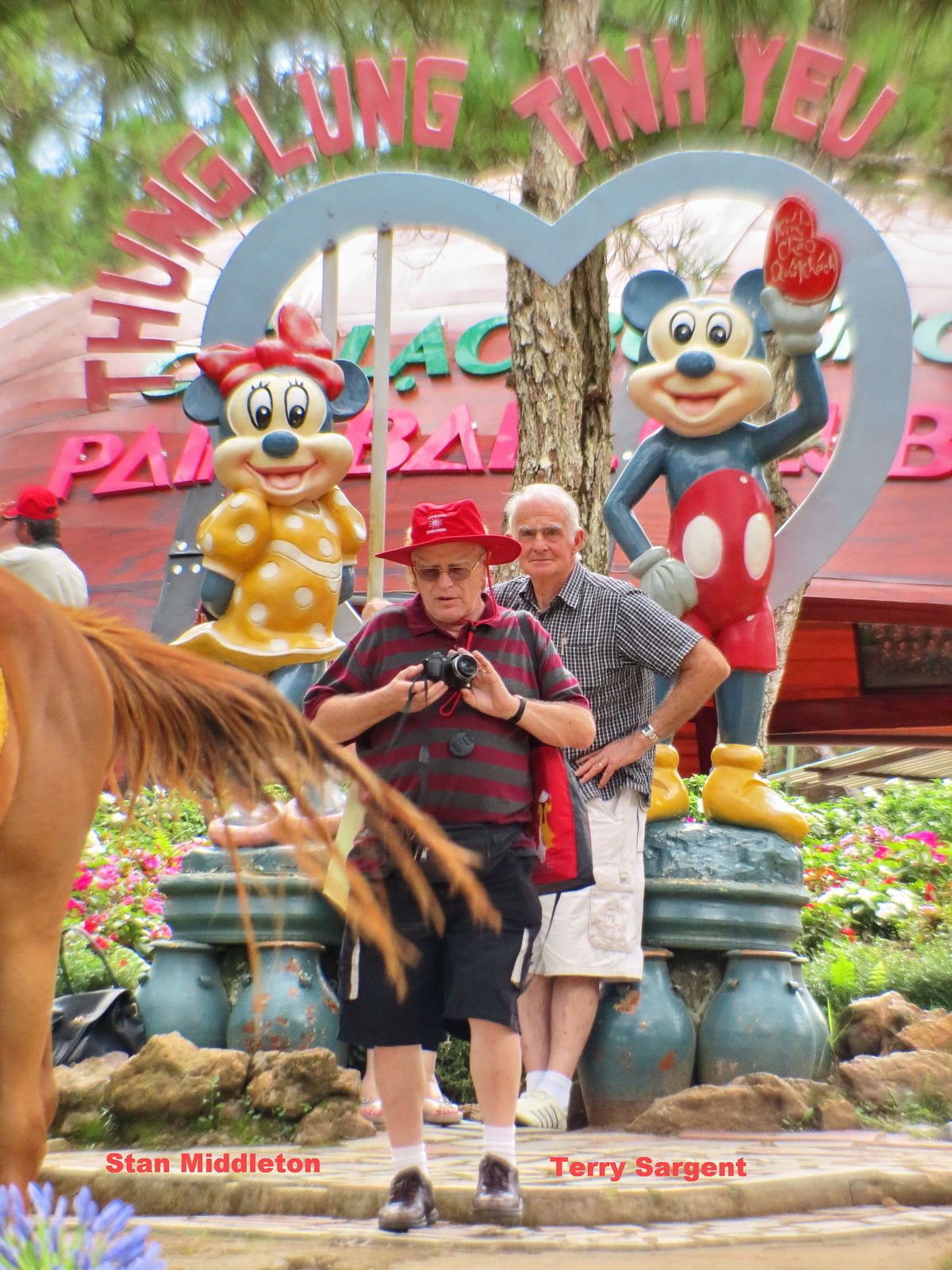This photograph captures two older gentlemen posing in what appears to be an amusement park. The background shows lush green trees, the trunk of a tree, and a reddish building adorned with red and green letters in an unfamiliar, possibly Asian language. Central to the image is a gray heart statue featuring Mickey Mouse and Minnie Mouse characters, with red letters above them spelling out "Thung Lung Tin Yu." 

The man in the foreground wears a red and gray striped shirt, black shorts, a red wide-brim hat, sunglasses, and holds a black camera. To his left, the other gentleman is dressed in a striped gray shirt, white shorts, and white shoes, leaning casually against the statue. Their names appear at the bottom of the photo in red text: "Stan Middleton" on the left and "Terry Sargent" on the right. Additionally, the left edge of the image reveals a partial view of a brown horse’s backside. Behind the men and the statue, you can see green plants, flowers, and a building with a circular-shaped roof further enveloped by tree branches.